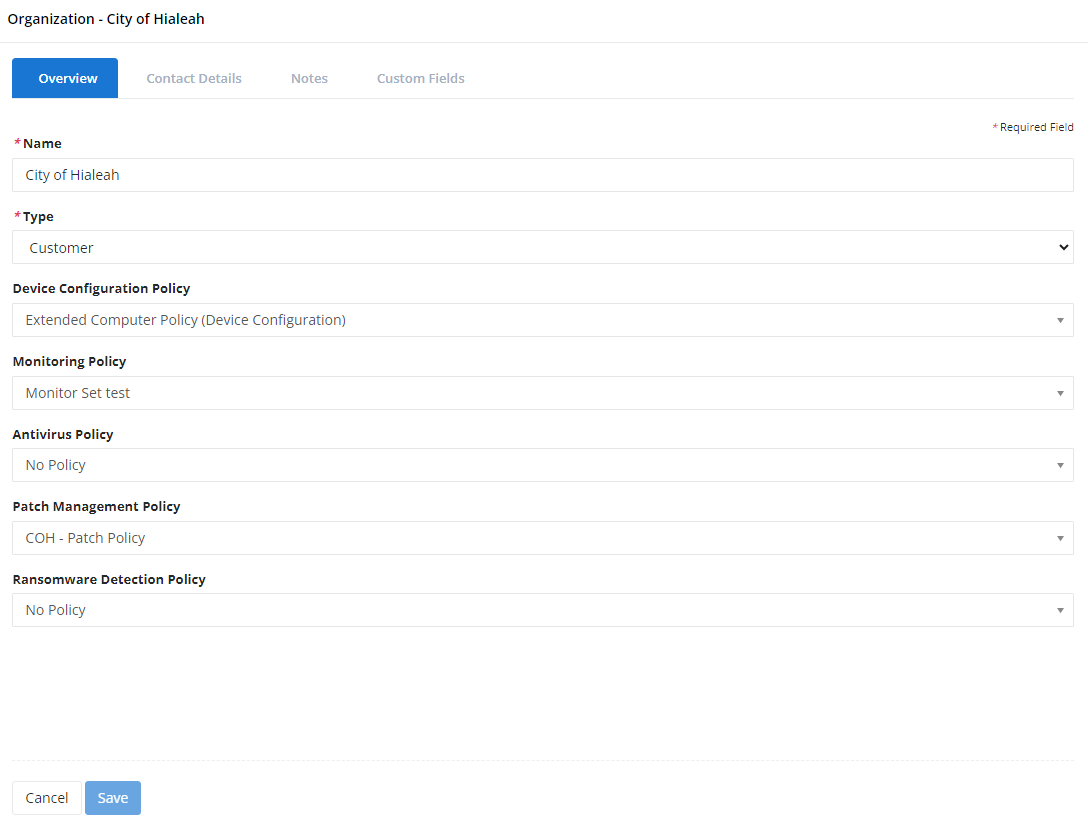The image depicts a user interface containing detailed information about an organization's configuration. At the top left, it indicates the organization as "City of Hialeah." Below, a blue rectangular box with the white text "Overview" is present. To the right of this box are several tabs labeled "Contact Details," "Notes," and "Custom Fields."

Underneath these headers is a field labeled "Name," marked with a red asterisk to denote it as a required field. The text field contains the value "City of Hialeah." 

Following that, a field labeled with an asterisk "Type" is set as "Customer." The next field is "Title," which reads "Device Configuration Policy" (not marked with an asterisk), and shows details such as "Extended Computer Policy" with "Device Configuration" in parentheses. Subsequent fields include "Monitoring Policy" set as "Monitor Set Text Test," "Antivirus Policy" with the value "No Policy," "Patch Management Policy" amply filled with "COH - Patch Policy," and finally, "Ransomware Detection Policy" also marked as "No Policy."

At the end of the row on the right, each entry field contains drop-down boxes for additional options.